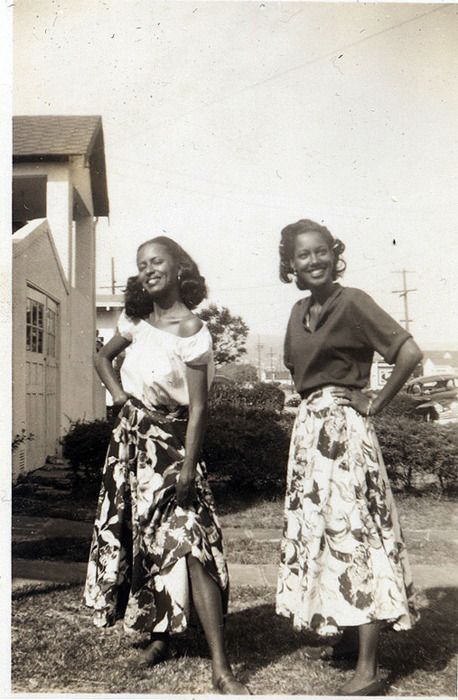This vintage black-and-white photograph, likely from the 1950s or early 1960s, features two smiling, happy African-American women standing on a lawn in front of a row of closely spaced stone or brick houses. To their left is a tall white house with a white garage, characterized by windows at the top of the door and a peaked roof. The background shows a hedge dividing the properties and possibly a parked car in the distance.

The woman on the left, who has long hair and brown skin, is wearing a white off-the-shoulder, short-sleeve blouse paired with a black-and-white floral ankle-length skirt. She playfully lifts her skirt with her extended left leg, revealing her shin up to the knee, and is wearing sandals. 

The woman on the right, slightly older with black hair and brown skin, is dressed in a dark mid-length sleeved sweater adorned with a neckerchief, and a white floral mid-calf print skirt. She stands facing the camera with her hands on her hips, also smiling. The shrubbery and row of houses in the backdrop amplify the vintage charm of this well-lit and lively scene.